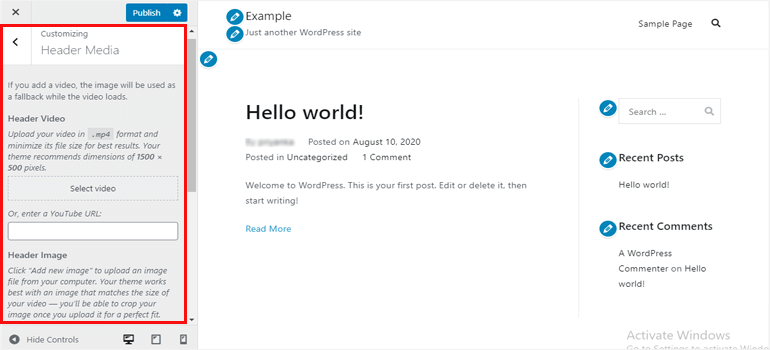**Caption:**

This image is a horizontal screenshot depicting the WordPress customization interface, predominantly showcasing the "Customizing Header Media" section. The interface is colored in shades of white, blue, red, and gray. On the left-hand side, a column is outlined with a thin red box, labeled "Customizing Header Media." Below this title, brief descriptions for "Header Video" and "Header Image" are provided, alongside options to select a video or enter a YouTube URL. At the bottom of this section are various controls and icons. A prominent blue "Publish" button with white text is situated at the top of the left-hand column.

The main portion of the screen exhibits a sample design for a WordPress site. The top-left corner displays "Example, Just Another WordPress Site." Below, in black text, the content reads "Hello World," posted on August 10, 2020, listed under "Uncategorized" with one comment. The introductory text states, "Welcome to WordPress. This is your first post. Edit or delete it, then start writing." A "Read More" link follows this text.

On the right side of the page, separated by a subtle vertical light gray line, is a search bar. Below the search bar are sections for "Recent Posts" and "Recent Comments." In the bottom right-hand corner of the interface, the text "Activate Windows" appears in a very light gray color.